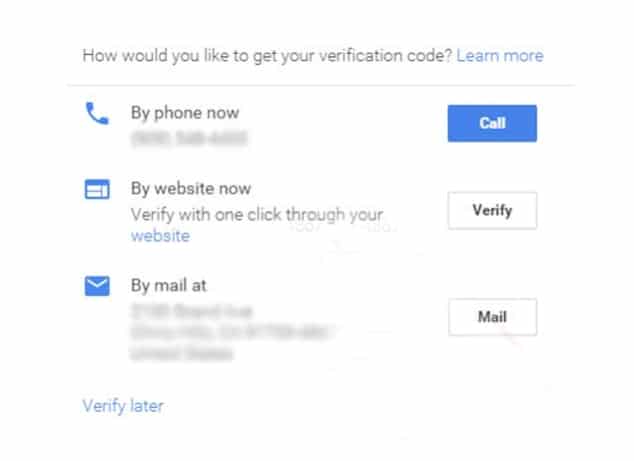This image depicts a computer screen displaying a section of a webpage concerning the retrieval of a verification code. At the top of the page, there is a prompt in gray text asking, "How would you like to get your verification code?" immediately followed by a blue hyperlink labeled "Learn more." 

Directly below this, a faint gray line separates the question from the options provided, which are arranged in distinct blue rectangles. 

The first option includes a blue phone icon with the text "By phone now." The associated phone number is blurred for privacy, and this option has a blue button on the right labeled "Call" in white text.

The second option is contained within a blue square and reads "By website now" with a subtext stating, "Verify with one click through your website," where the word "Website" is a clickable blue link. The blue rectangle on the right has a black button that says "Verify."

The third option features a blue envelope icon alongside the text "By mail at," with the mailing address obscured for privacy. This section includes a button labeled "Mail" at the end of the line, and below this, there is an option to "Verify later" in blue text.

This detailed layout provides multiple methods for users to receive and verify their code.